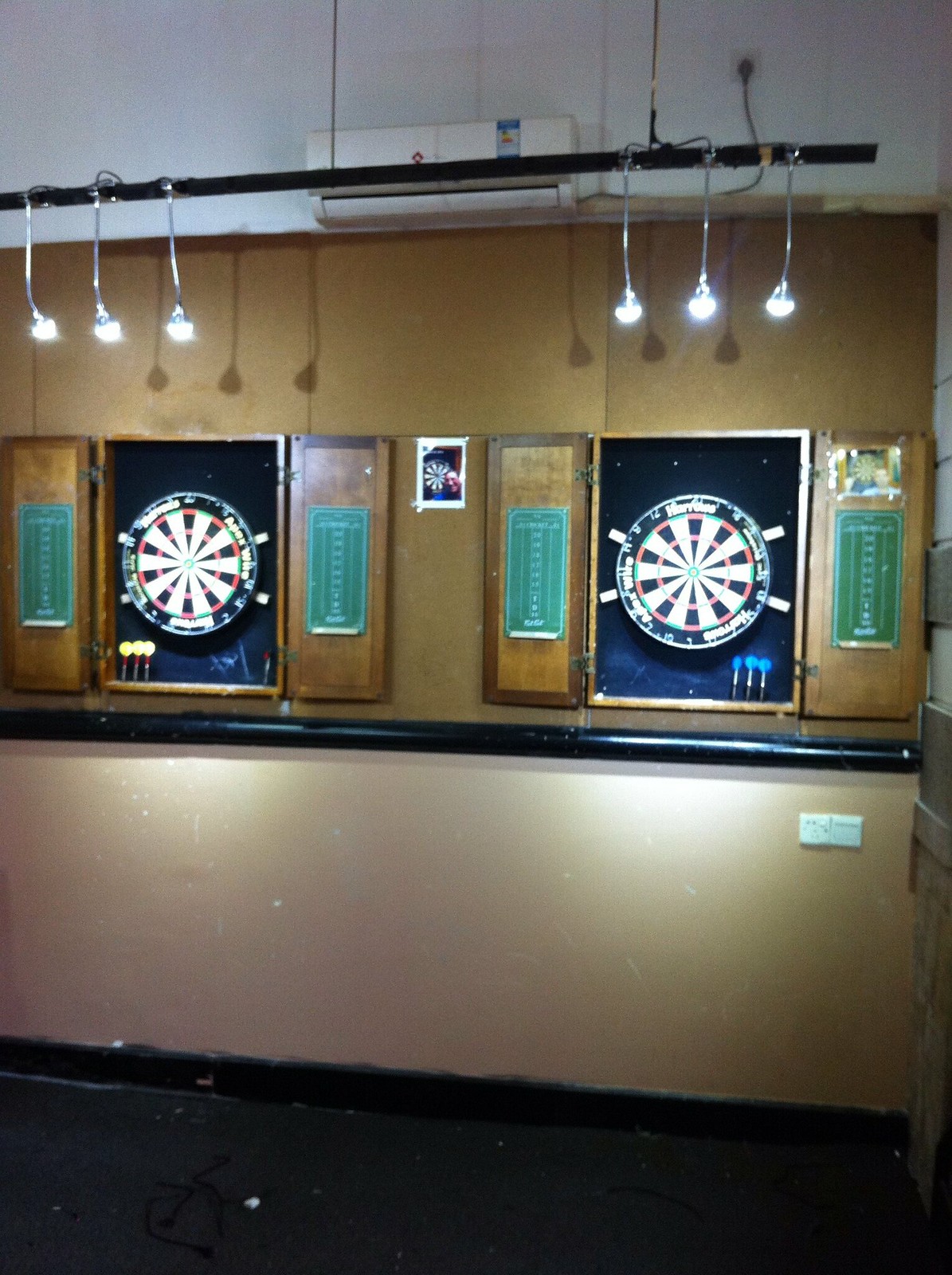This image depicts a game room featuring two dartboards housed in cabinets mounted on a light brown wall. The dartboard cabinets include dark blue backdrops and light brown wooden frames with green chalkboard panels inside each door for scoring. Positioned at the top of the image is a row of track lighting that illuminates each dartboard with three pendant lights, creating shadows on the wall above. Additionally, a white heat pump is mounted near the ceiling. Each dartboard is equipped with three darts, blue on the right and yellow on the left. Below the dartboards is a black chair rail and a matching black baseboard outlining the base of the darker floor. The lower half of the wall contrasts in a lighter brown tone. On the lower portion of the left cabinet door hangs a picture framed in white, depicting another dartboard. A light switch is visible near the floor beneath the dartboards.